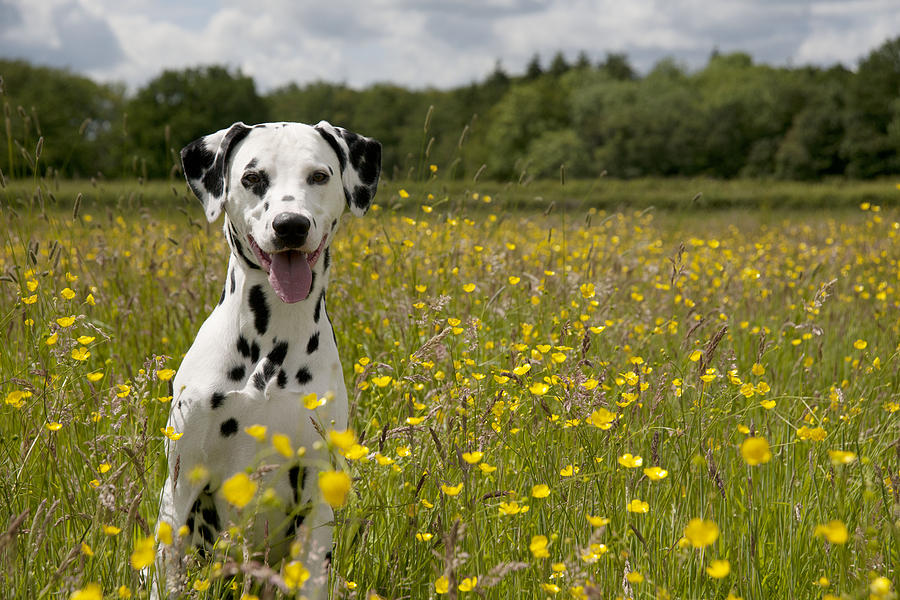In this vibrant full-color photograph, a cheerful Dalmatian, predominantly white with distinctive black spots, stands out against a picturesque natural setting on a partly sunny day. The scene is captured using natural light, with the upper portion of the image dominated by clouds, leaving little visible blue sky. Stretching across the background, a distant blur of trees and an open field creates a serene, untouched backdrop.

The lower half showcases a more focused view of a lush field teeming with small, yellow flowers, reminiscent of daisies, that bloom proudly among the green grass. The Dalmatian is positioned off-center to the left, facing the camera with a friendly, open-mouthed smile and a pink tongue hanging out, conveying an energetic and playful demeanor. The dog’s floppy ears and bright expression suggest a youthful vitality, even if it might be a fully grown dog. The overall composition emphasizes the harmony of the natural elements, with no visible human-made structures, highlighting the beauty and tranquility of the outdoors.